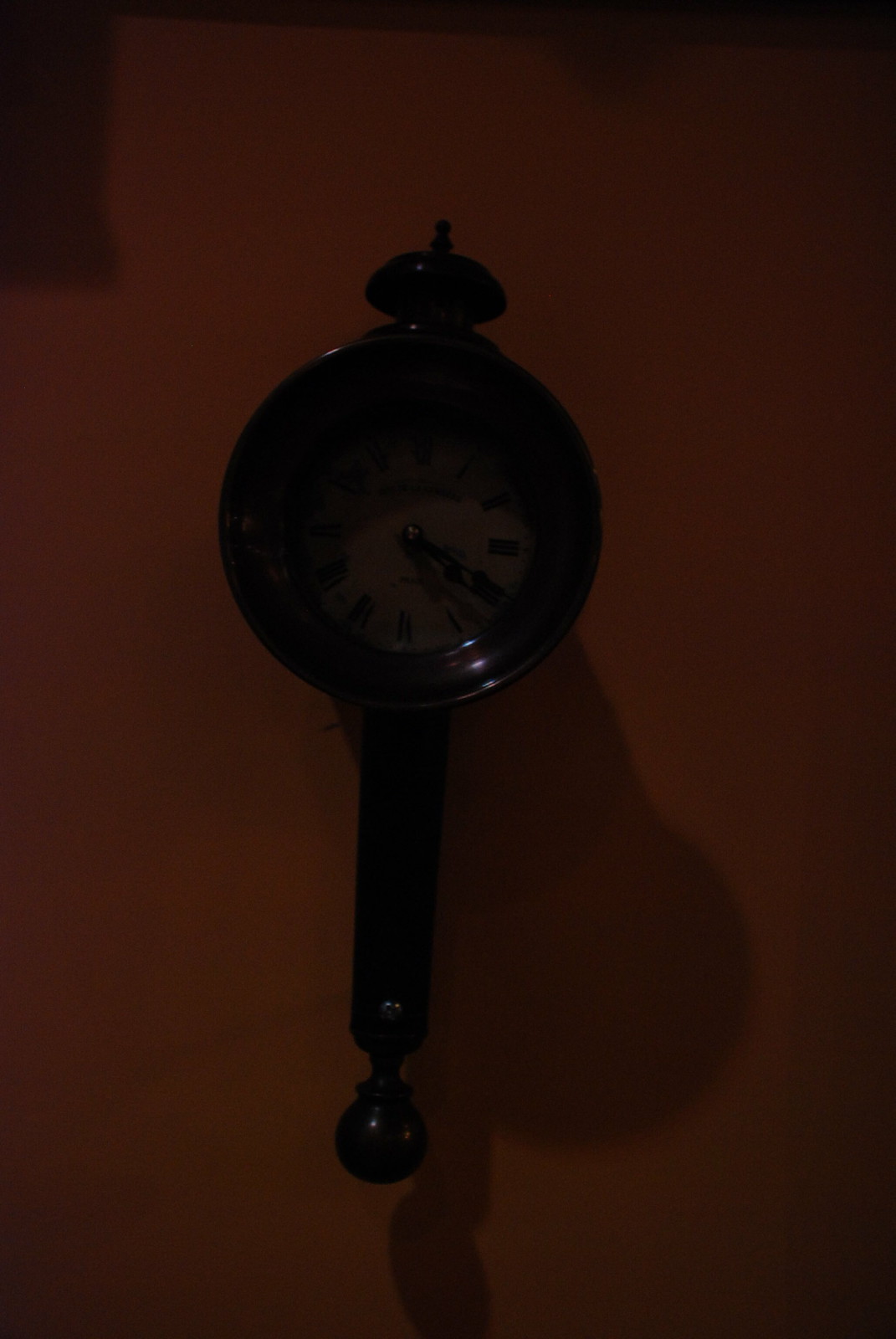This photograph features a wall-mounted clock set against an orange-toned background, which leans towards a deep, almost brownish hue. The dim lighting of the scene casts shadows and subtle highlights, creating a somewhat mysterious ambiance. The clock itself boasts an elegant wooden frame made from a rich, dark wood. Its design is reminiscent of a traditional tabletop bell, with a distinct cylindrical portion that gracefully extends downward, ending in a decorative wooden ball. The clock's face is a stark white, standing out against the darker surroundings. Roman numerals from I to XII encircle the face, clearly marked in black, mirroring the color of the clock’s hands.